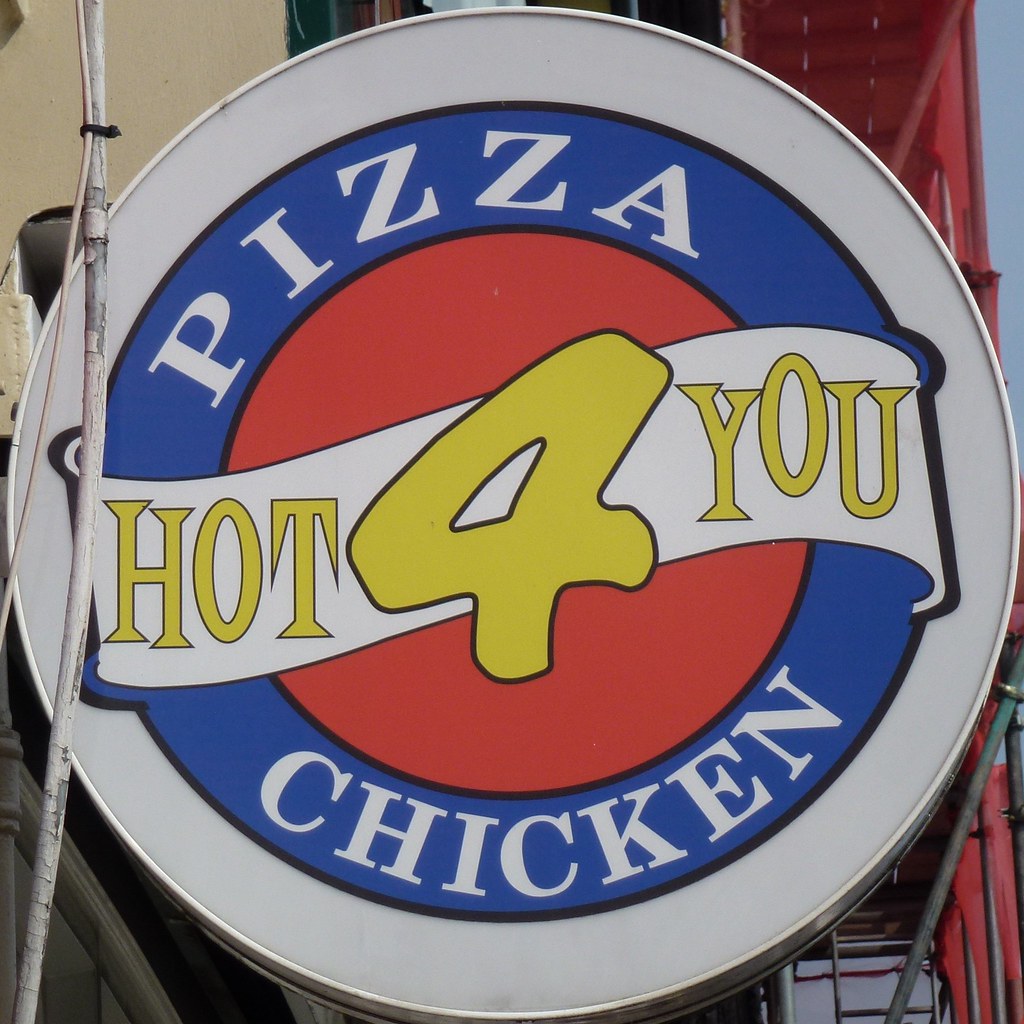The image depicts a large, circular logo for a pizza shop, prominently featuring bold colors and text. The outermost section of the logo is a white border, followed by a concentric blue circle. Within the blue circle, "pizza" is written in large white letters at the top, and "chicken" is similarly displayed at the bottom. At the center of the logo is a red circle, over which a white banner stretches horizontally. On this banner, the phrase "hot 4 you" is written in yellow, with the number "4" notably larger than the rest of the text. The image appears to be taken outdoors and is heavily zoomed in, making the surroundings somewhat obscure. However, visible details include several metal poles and wires intersecting in front of the sign. Behind the logo, there are indications of construction work, with structures resembling ladders and stairs, as well as a mix of a beige wall, a red awning or covering, and glimpses of blue sky and additional red material, possibly curtains, on the edges.